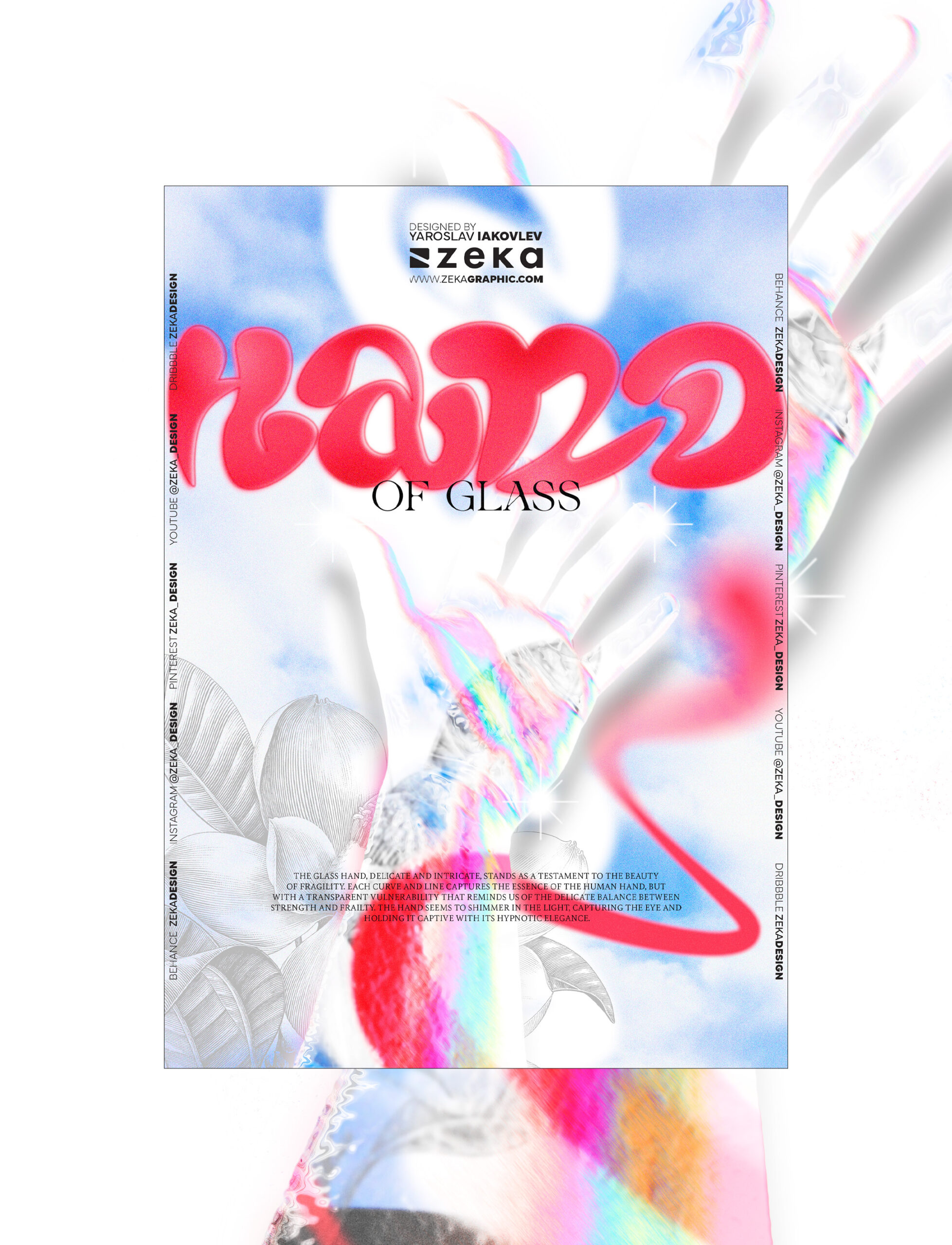The image depicts a highly stylized front cover, likely of a magazine, featuring a sky-blue background with various abstract details. Central to the design is a reflective glove that displays an array of iridescent hues including purples, pinks, yellows, and blues. This glove appears almost like a fish due to its shimmering qualities. The main text at the top reads "Hand of Glass" in a decorative red font, with "of glass" being in smaller black text beneath it. 

Designed by Yaroslav Iakovlev, the cover bears the branding of Zeka, denoted by its logo and the website www.zekagraphic.com. The background extends into a complex pattern featuring leaves and spirals, further enhancing the abstract theme with reds, blues, and whites. Additional small, slanted text appears on both sides surrounding a larger, blown-up image of the reflective glove, contributing to the intricate and detailed visual appeal. At the bottom of the page, there's a paragraph, supplementing the visual elements with textual information.